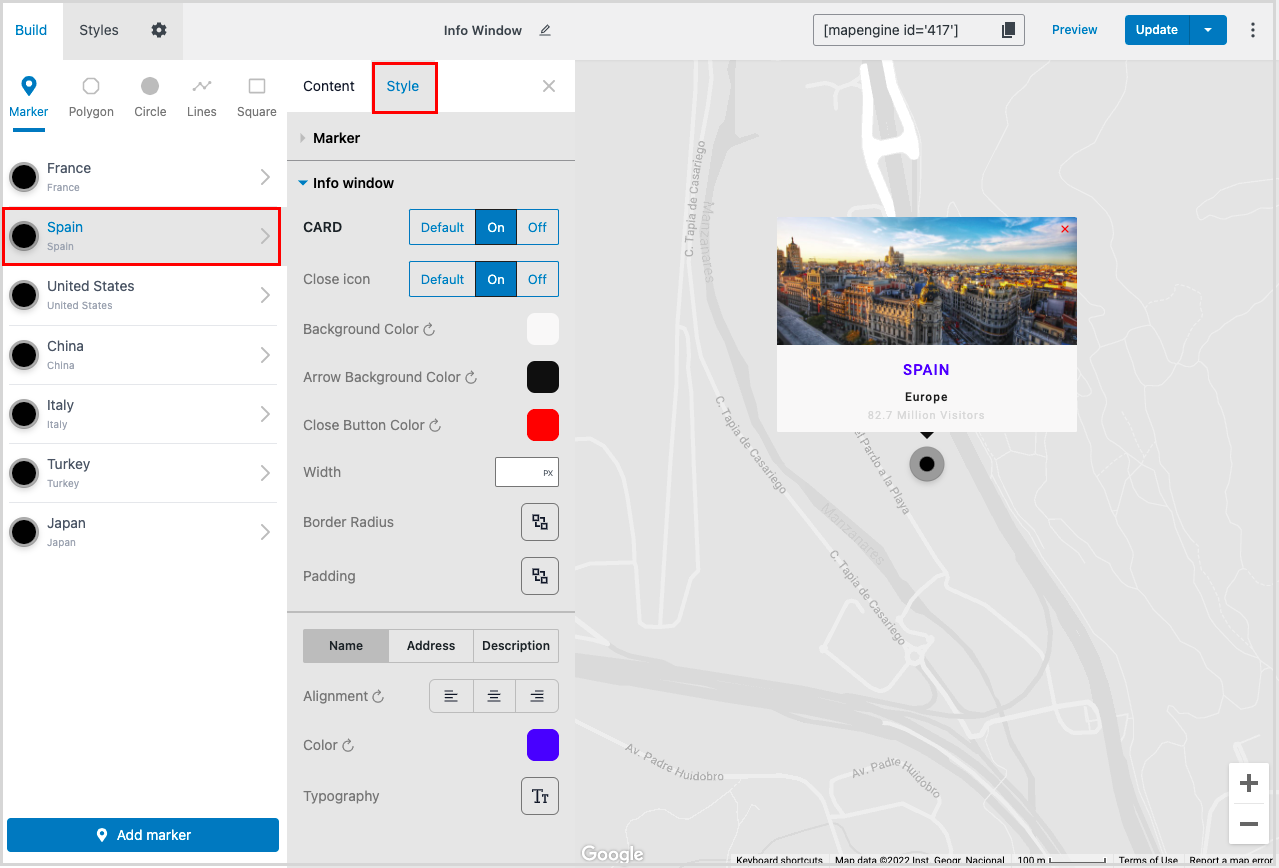A detailed photo of a map-building website interface. 

On the left, the "Build" tab is selected, displaying various tools such as Marker, Polygon, Circle, Line, and Square. Below this, a list of countries is provided, including France, Spain, United States, China, Italy, Turkey, and Japan, each with a right arrow indicating further options.

Towards the center, the "Content" tab is visibly blacked out, while the "Style" tab is highlighted in blue and surrounded by a red rectangle. Beneath the "Style" tab, a blue rectangle button labeled "Add Marker" is prominently displayed. 

The detailed options under the "Style" tab are explicitly shown: "Marker" and "Info window" with a blue downward arrow indicating it has been expanded. Options within this section include "Card" (default on, currently on), "Close icon" (default on, currently on), "Background color" (white), "Arrow background color" (black), "Close button color" (red), and a blank box for "Width". Further fields like Border radius, Padding, Name, Address, Description, Alignment, Color, and Topography are also listed.

To the right of this interface section is a map featuring zoom controls (plus and minus signs for zooming in and out). The map shows Spain in Europe, alongside a statistic indicating millions of viewers. Additionally, there is a clickable rectangular thumbnail showcasing an image of downtown Spain.